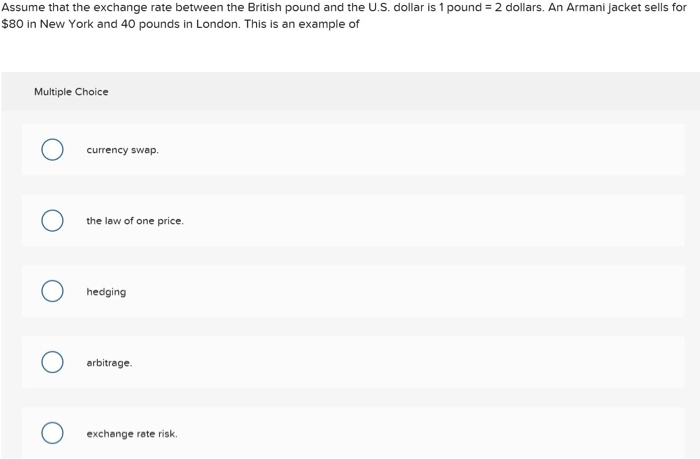Screenshot on a white background showcasing a multiple-choice question related to exchange rates and pricing. The question states: "Assume that the exchange rate between the British pound and the US dollar is one pound equals two dollars. An Armani jacket sells for $80 in New York and 40 pounds in London. This is an example of:" Below the question, there's a light gray box with the title "Multiple Choice" at the top. The box contains five options, each marked by a white circle with a dark blue border. The options are:

1. Currency Swap
2. The Law of One Price
3. Hedging
4. Arbitrage
5. Exchange Rate Risk

The entire content is neatly organized, but the answer to the question is not provided.